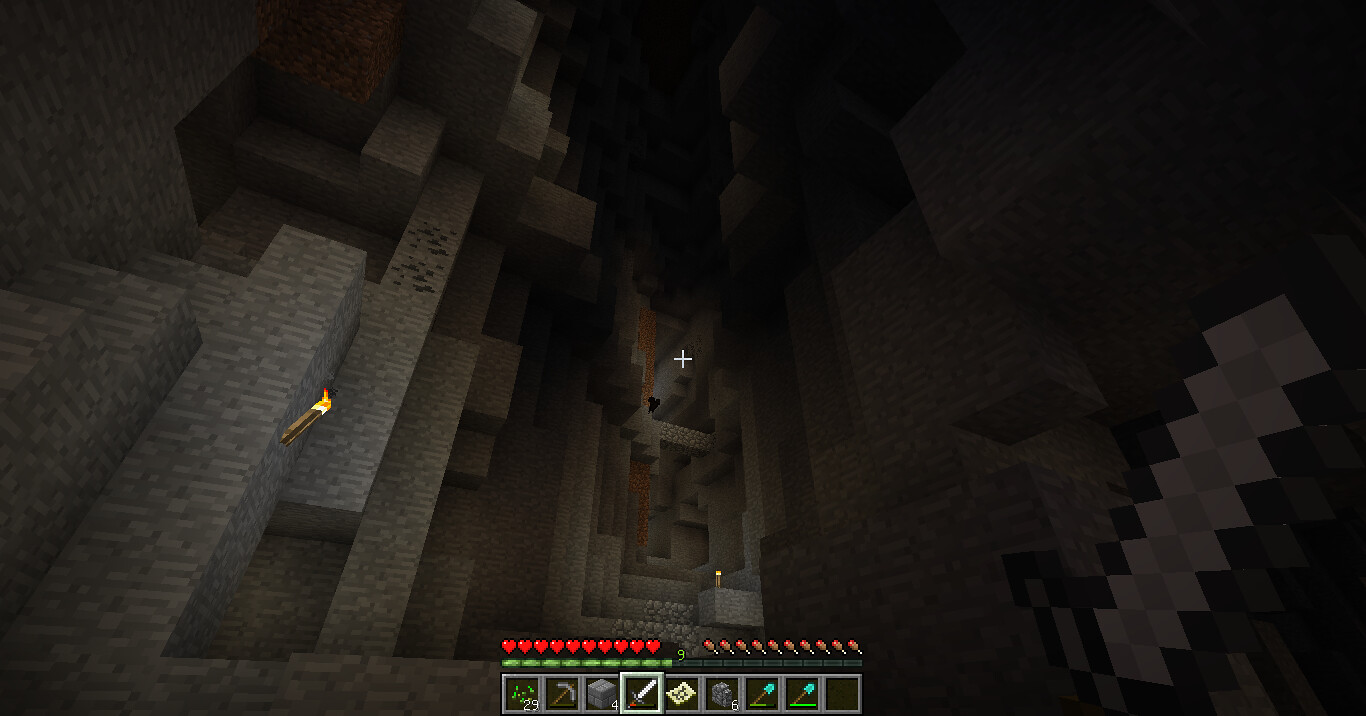The image is a detailed screenshot from the game Minecraft, captured from a first-person perspective. The setting is an expansive, dark cavern characterized by the game's iconic blocky, voxel graphics. The cavern's upper right corner fades into an extremely dark charcoal gray, contrasting with the light brown and mottled darker gray stones that dominate the rest of the scene. The cavern appears to be filled with long stone columns, possibly arranged both upright and piled on top of one another, especially dense on the left side of the image.

In the center, these columns form a stair-like structure, hinting at a passageway that might lead to a dungeon-like area. A distinct light brown zigzag-shaped object traverses diagonally from the bottom toward the top right. The top section contains coal blocks, and the entire scene is subtly illuminated by torches.

At the bottom of the image, the heads-up display (HUD) is visible. It shows the player's health, nearly full, and hunger meter, indicating they are well-fed. The time meter, possibly green, alongside the inventory, reveals a pickaxe, an iron sword held in the character’s right hand, and two diamond spades among other items. Additionally, tiny icons display power levels and other gameplay metrics, though they are too small to discern clearly. On the left side above these icons, a series of red hearts can be noticed, while on the right, tiny flower-like symbols are visible.